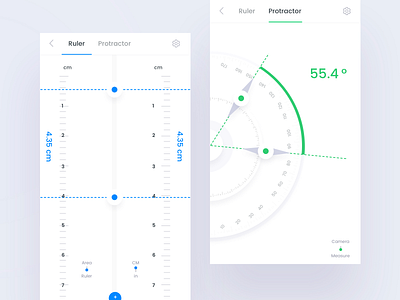This photo features a digital measurement tool app or website with a gray background, displaying both a ruler and a protractor. On the left side, a white ruler with blue details marks centimeters from 1 to 7, with an emphasis on the measurement of 4.35 centimeters indicated by blue dotted lines and text. The right side showcases a white protractor, highlighted in green, with green dotted lines illustrating its measuring capability. The protractor is marked with the angle 55.4 degrees in green text. The clear visual separation and distinct colors used for measurements (blue for the ruler, green for the protractor) enhance usability and clarity in understanding how each tool functions.